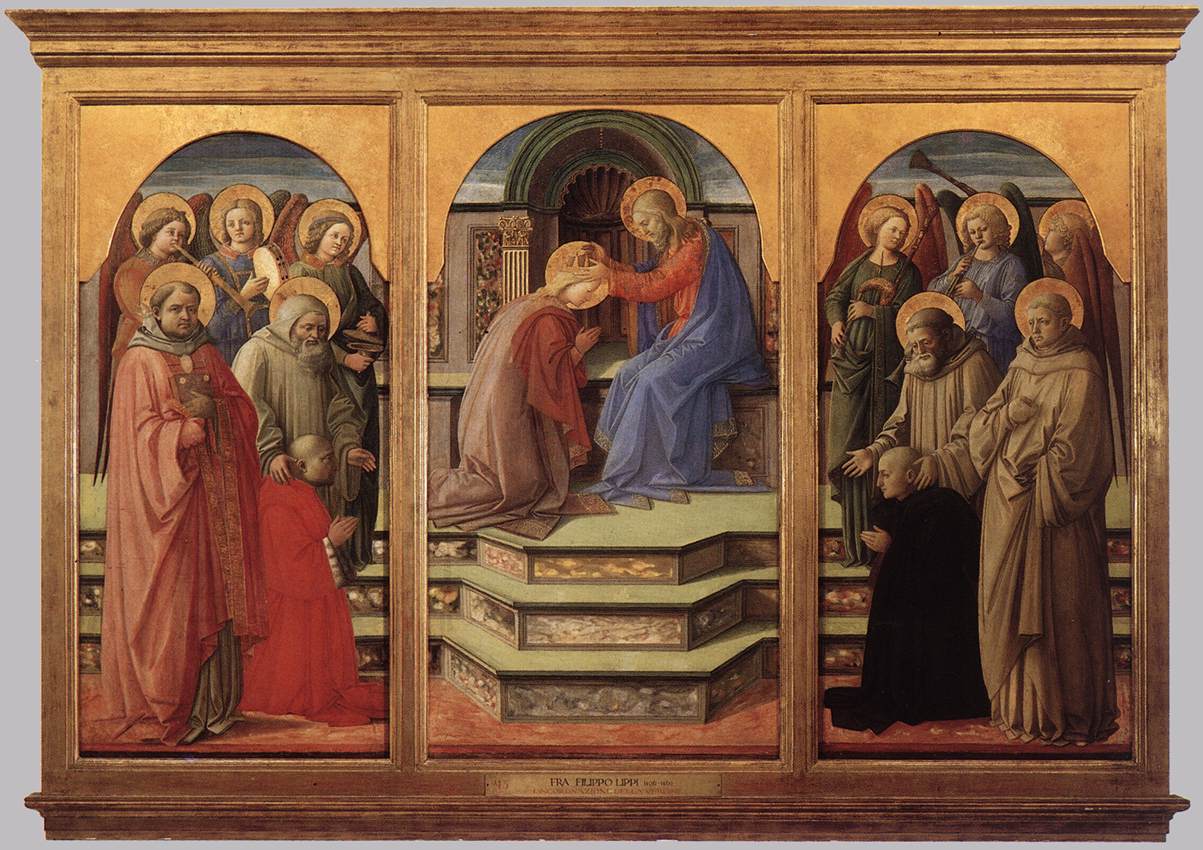The image is a detailed diorama housed within a goldish brown wooden cabinet, partitioned into three open sections: left, middle, and right, each topped by a small bronze archway. Below the middle section, there is a central plaque that partially reads “Filippo Lippi,” though the rest of the writing remains unclear.

In the left section, there is a group of six people. The central figure is a bald man in a red gown, kneeling. Surrounding him are two men and three women, each with golden halos around their heads. The women appear to be playing musical instruments.

The middle section features three green steps leading up to a platform. A figure that strongly resembles Jesus sits on the right, adorned in a blue cloak and red garment, extending his hands towards a kneeling person on the left, appearing to bless or crown them. This central figure reinforces the sense of a sacred or holy scene.

The right section mirrors the left with another group of six people. The central kneeling figure wears a black gown, accompanied by two men and three women behind him, who are also playing musical instruments and have golden halos.

All the figures, with their halos and sacred postures, suggest this triptych portrays a biblical or saintly narrative, focusing on a Christ-like blessing in the middle, observed by groups of revered individuals on either side.